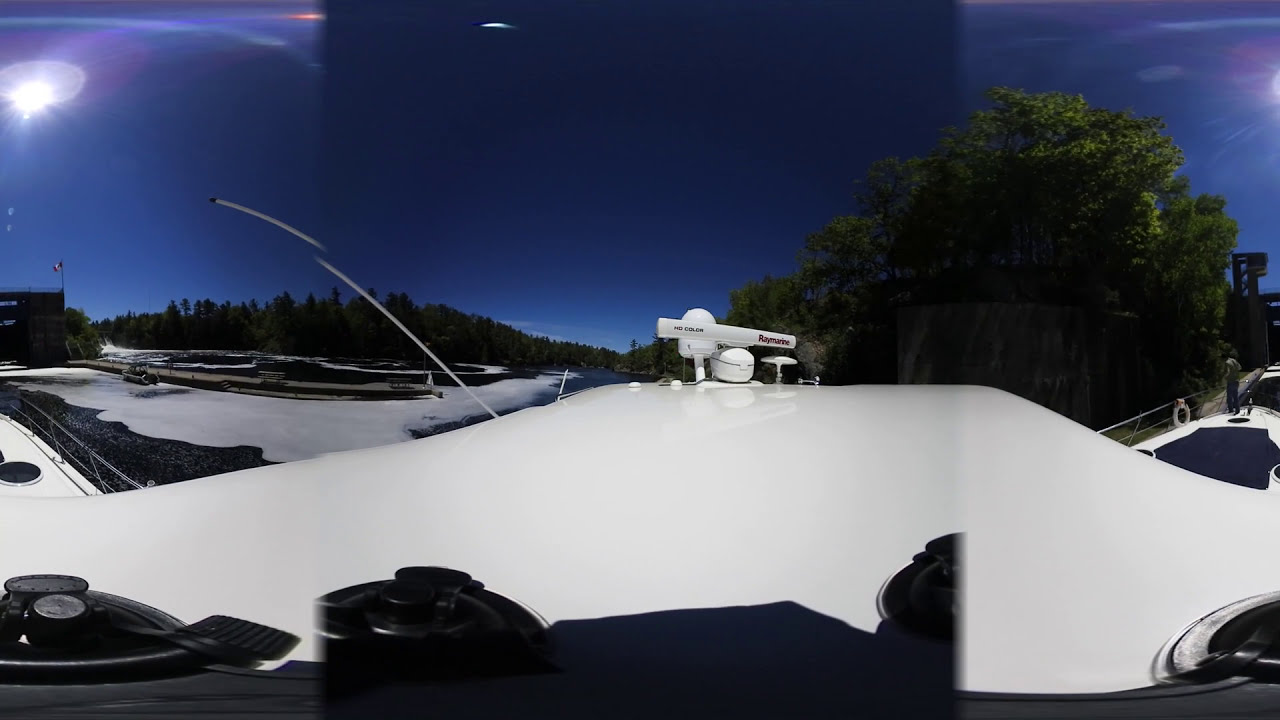In this image, the sky occupies the top half, predominantly a very dark blue with a lighter, brighter blue on the right. In the left upper corner, there's a light source resembling the Sun. Below the sky, a dense bank of green trees stretches across the horizon, punctuated by a taller tree with visible leaves on the right. In the middle-left, there is a building flying what appears to be the Canadian flag. 

The midsection shows a river with white streaks suggestive of a waterfall or rapids. This leads into the foreground, where the image appears distorted. Here, the scene depicts the roof of a boat, creating an almost stitched-together effect with unusual angles and proportions. The boat’s roof is white, housing various pieces of equipment, including a round object and a tall, rectangular object resembling GPS antennas. Silver railings are visible on both the left and right sides of the boat. 

Overall, the setting is outdoors with a mixture of blue, green, white, and silver colors, suggesting an environment with trees, water, and a vehicle—most likely a boat.